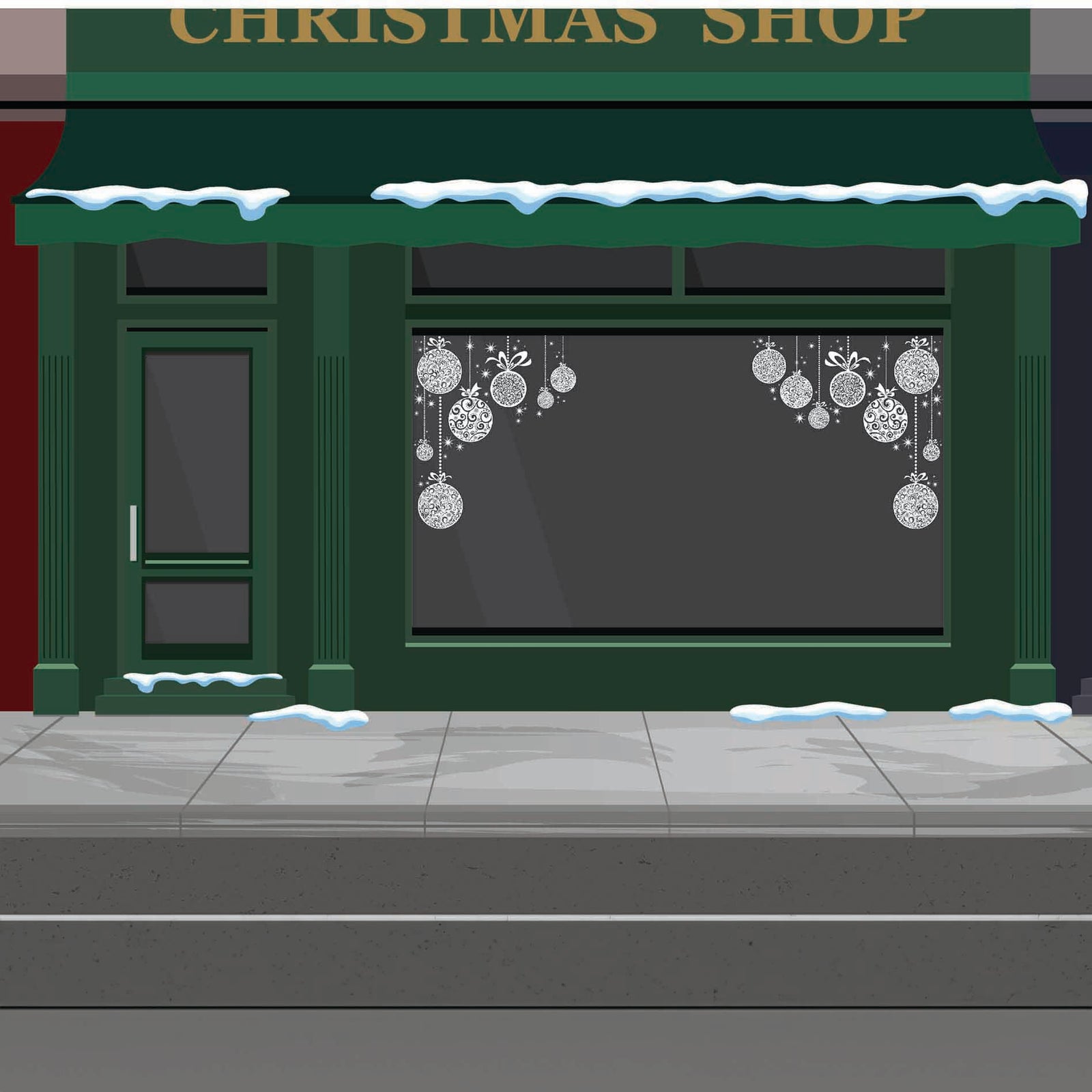This digital rendering portrays a quaint Christmas Shop with meticulous detail. At the top, partially cut off, the green sign reads "Christmas Shop" in gold lettering. Snow dusts the ledge above and the awning edge. The storefront is painted a festive green, with a single door to the right and a large display window to the left. The door, slightly gray in its center, is approached by steps dusted with snow. The window features white-drawn Christmas ornaments with sparkles, set against a gray and green background. Patches of snow sprinkle the gray concrete sidewalk that lines the street, which is marked by a white dividing stripe. This charming scene captures the essence of the holiday season in a digitally illustrated townscape.